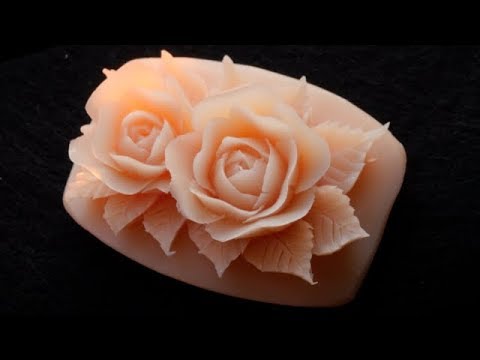The image showcases a highly detailed, handcrafted bar of soap set against a completely black background, which draws all attention to the intricately made product. The soap itself is a light pink, salmon skin color, presenting an elegant and luxurious appearance. Carved into the top of the bar are two exquisite 3D roses, each with intricate petals and veins, meticulously detailed to appear lifelike. The roses are about half-opened, adding to their realistic look and the delicate craftsmanship. Surrounding the base of the roses are equally detailed leaves, further enhancing the natural aesthetic. There is no packaging or branding visible, making it a clean and focused product shot, possibly intended for a high-end soap brand or an advertisement for luxury handmade soaps. The subtle lighting highlights the meticulous carvings, adding depth and emphasizing the bar's artistic quality.